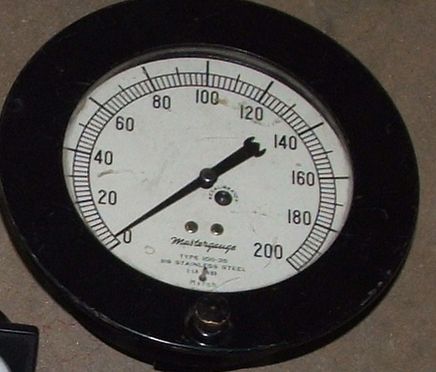The image features a brownish-gray background. In the lower left-hand corner, there is a black object with a small white section at its corner. At the center of the image, there is a prominent, thick black circle containing a smaller nut-like structure at its base. Within the black circle, there's a white inner circle with numerical markings and longer lines indicating the numbers, which range from 0 to 200 in increments of 20 (0, 20, 40, 60, 80, 100, 120, 140, 160, 180, 200), and shorter lines in between. A single arm or pointer, featuring three points—one on each side and a triangular shape in the middle—extends near the zero mark. The arm passes through a couple of small metal circles. Above one of these metal circles, there is some writing that is too small to discern, and similar indecipherable writing is positioned below the metal circles as well.